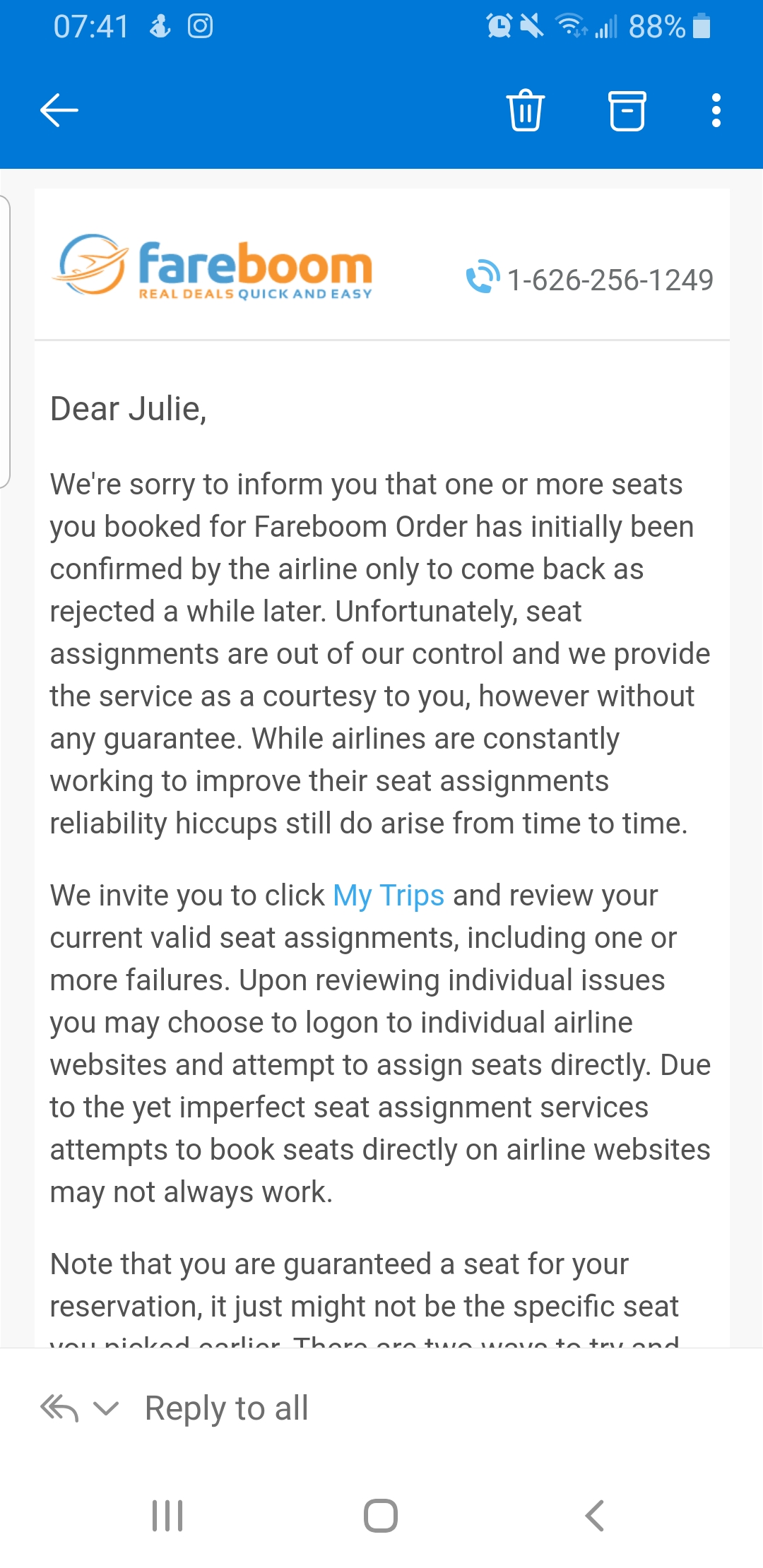**Caption:**

This image is a detailed screenshot of a message received through the Fareboom app on a smartphone. The screen predominantly features a white background with black text and various interface elements. At the top of the screen, a blue bar displays the phone's information, showing the time as 7:41 AM, along with icons indicating a fitness notification, an Instagram notification, an active alarm, muted sound, Wi-Fi connectivity, half cell service, and an 88% battery charge.

Inside the app interface, several icons are visible, including a back arrow to navigate to the main message page, a trash can icon to delete the message, an archive icon, and three vertical dots for more options. The top of the message includes the Fareboom logo, featuring blue and orange text that reads "Real Deals, Quick and Easy," accompanied by their logo. Beside this is a presumed customer service phone number: 1626-256-1249.

The message itself addresses a user named Julie and informs her that seats initially confirmed for her Fareboom order were later rejected by the airline. It emphasizes that seat assignments are controlled by the airline and, despite efforts, discrepancies can occur. A blue hyperlink labeled "My Trips" invites Julie to review her current valid seat assignments. The message advises her to log onto individual airline websites if she wishes to attempt seat assignments directly, though it notes that these attempts may not always be successful. It reassures Julie that she is guaranteed a seat, although it may not be the specific one she initially chose. The message's final line is cut off and unreadable.

At the bottom of the screen, there are options to reply, indicated by a back arrow, and a drop-down arrow beside "Reply to all." Standard phone control buttons—back and minimize—are located in the bottom menu.